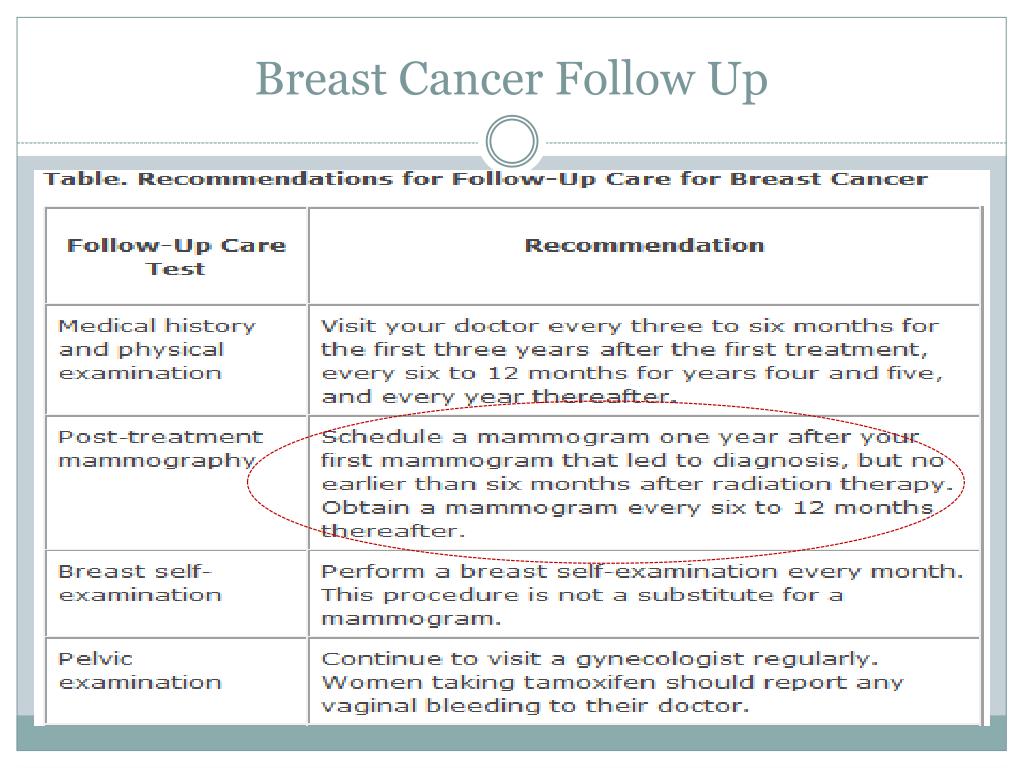The image features a white background with a faint blue borderline, resembling a table format. At the top, in faint blue text, the words "Breast Cancer Follow-Up" are written. Below this heading, there's a title in black ink, "Table: Recommendations for Follow-Up Care for Breast Cancer."

The table is composed of two columns and several rows, detailing various follow-up care tests and recommendations:

1. **Medical History and Physical Examination**: 
   - **Recommendation**: Visit your doctor every three to six months for the first three years after initial treatment, every six to twelve months during years four and five, and annually thereafter.
   
2. **Post-Treatment Mammography**:
   - **Recommendation**: Schedule a mammogram one year after your initial post-treatment mammogram. The mammogram should be obtained no earlier than six months after radiation therapy and then every six to twelve months subsequently.
   
3. **Breast Self-Examination**:
   - **Recommendation**: Perform a breast self-examination monthly. Note that this is not a substitute for a mammogram.
   
4. **Pelvic Examination**:
   - **Recommendation**: Continue regular visits to your gynecologist. Women taking Tamoxifen should report any vaginal bleeding to their doctors.

A red, dotted oval encircles a portion of the text, emphasizing important follow-up care details. All the text within the table is written in black ink.